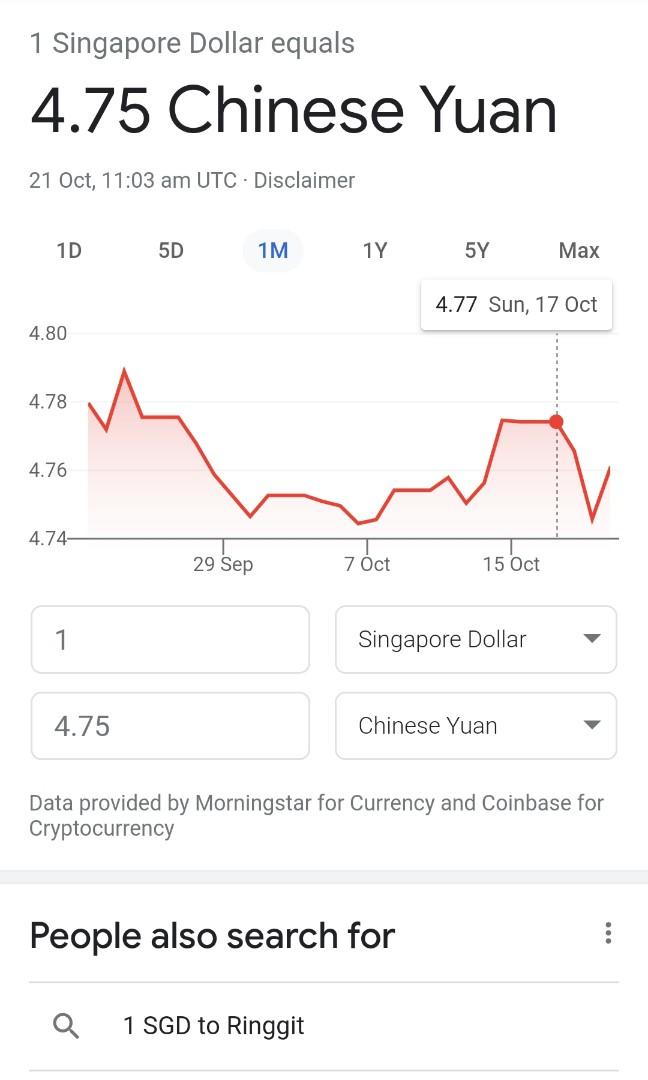### Detailed Caption

This image is a detailed screenshot from a financial application on a smartphone, displaying the exchange rate between the Singapore Dollar (SGD) and the Chinese Yuan (CNY). 

At the top of the screenshot, in dark gray text, it reads "One Singapore Dollar equals," followed by a prominently displayed "4.75 Chinese Yuan" in larger black text. Beneath this, in smaller gray text, there is a timestamp: "21st October, 11:03 a.m. UTC," accompanied by a disclaimer.

Just below this text, a navigation bar provides various time frame options for viewing the exchange rate trends: "One Day," "Five Days," "One Month," "One Year," "Five Years," and "Max." The "One Month" option is currently selected, highlighted in blue text on a light gray background.

A chart dominates the middle part of the image, with days marked along the x-axis and exchange rate values on the y-axis, ranging from 4.74 to 4.80. A specific data point on the chart is highlighted, showing "4.77" with a tooltip indicating the date as "Sunday, 9th October."

Below the chart, the interface displays conversion boxes in a two-by-two grid. The top-left box reads "1" and the top-right box reads "Singapore Dollar." In the bottom-left box, it shows "4.75" and the bottom-right box reads "Chinese Yuan."

At the bottom of the screenshot, two sources of data are credited: "Data provided by Morningstar for currency and Coinbase for cryptocurrency."

Further down, a section labeled "People also search for" appears, featuring a magnifying glass icon and the suggested search keywords: "1 SGD" and "2 RN GG IT."

This comprehensive screenshot encapsulates the real-time currency exchange data between the Singapore Dollar and the Chinese Yuan, as provided by a sophisticated financial application.